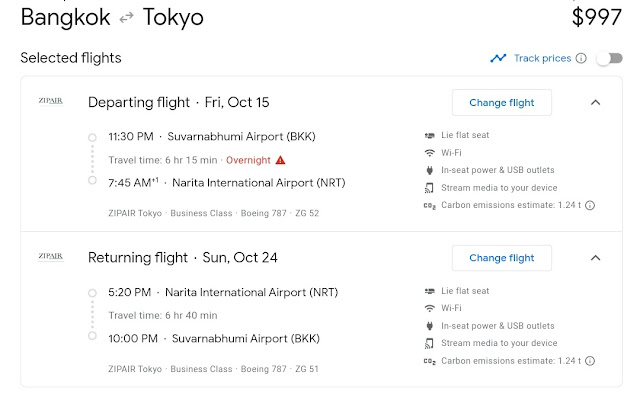Screenshot of Google Flights showing a round-trip flight from Bangkok to Tokyo priced at $997. The flight duration is approximately 6 hours and 15 minutes, which seems longer than expected for an intra-Asia journey. The airline listed is Zip Air, Japan's new budget airline known for its affordability. This fare strikes as quite high for the route distance. The image sparks interest in comparing prices for round-trip flights from Los Angeles to Tokyo, highlighting a desire to revisit Tokyo. Overall, it offers a glimpse into current airfare rates and travel options.